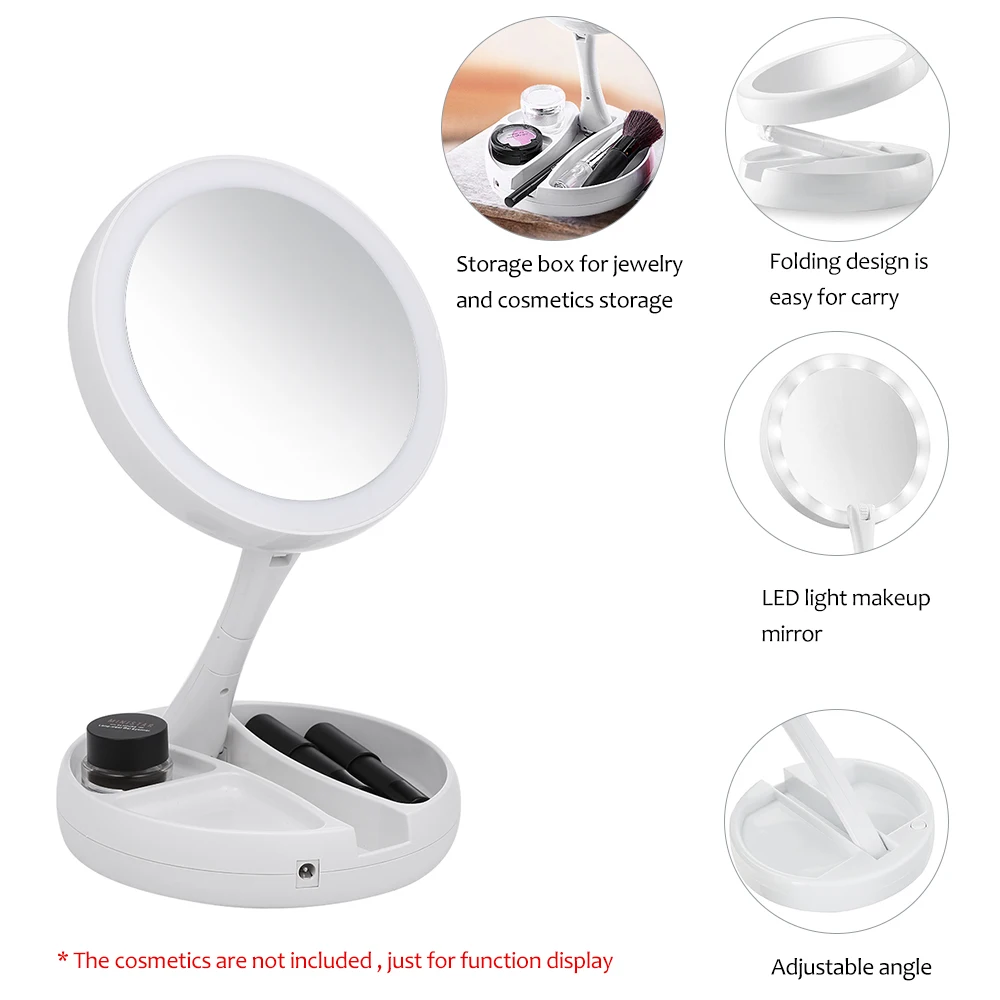This photo showcases an elegant beauty product designed for cosmetic storage. Presented in portrait orientation on a pristine white background, the central product features a circular base that lies flat on the surface. Mounted on the base are multiple small trays or compartments, providing organized spaces for various beauty items. 

Extending from the base is a stem-like apparatus supporting a circular mirror, which folds neatly into a designated recess in the base. The mirror, framed in white with a reflective gray surface, complements the overall white color scheme of the product. A power cord is visibly attached, suggesting the presence of an integrated light feature.

Within one of the compartments, a tiny glass jar and two pen-like tools are neatly placed, emphasizing the product's utility. The area beneath the mirror includes a note indicating that the depicted cosmetics are for illustrative purposes only and not included with the product.

To the right of the mirror, a colorful bubble highlights the product's capacity as a storage solution for both jewelry and cosmetics. Additionally, three smaller bubbles are aligned vertically, each describing a key feature of the product: 

1. Folding design for easy portability.
2. LED makeup light mirror for enhanced visibility.
3. Adjustable angle for customizable use during makeup application. 

The detailed layout and thoughtful design make this beauty product a practical and stylish addition to any vanity space.